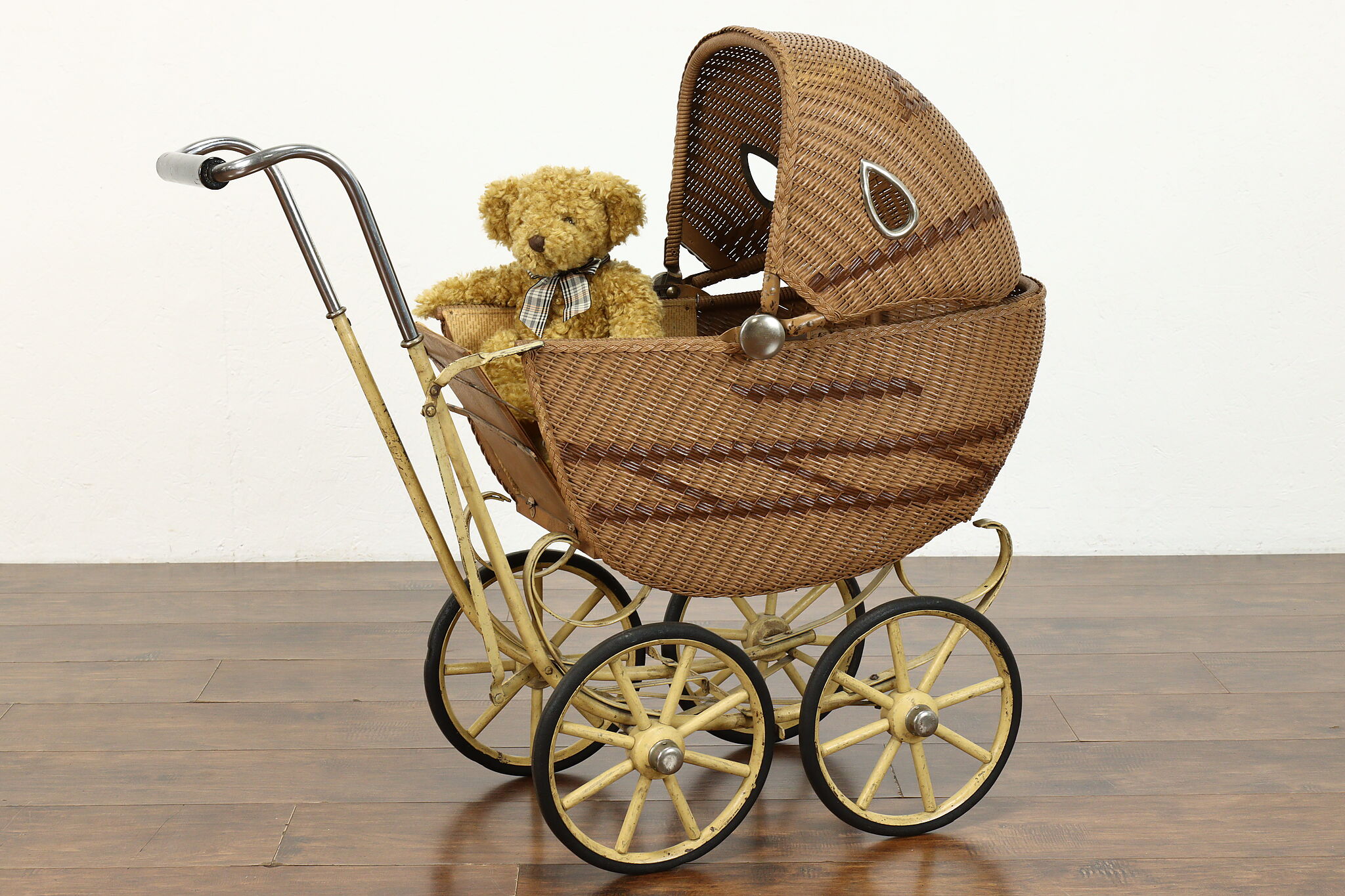This is a close-up photograph of a vintage wicker baby stroller, often referred to as a pram in England. The stroller, made from intricately woven wicker, features a hinged wicker hood that can be adjusted to provide shade and is attached with a prominent metal button. Seated inside the pram is a golden brown teddy bear adorned with a plaid tie. The stroller's frame, primarily metal with aged brass accents, has discolored over time. The handle, partially finished in tarnished chrome and off-white, is marked by its antiquity. The stroller's brass-spoked wheels, featuring thin black rubber tires, hint at its long history. The entire scene is set against a dark brown hardwood floor with a white wall serving as the backdrop.